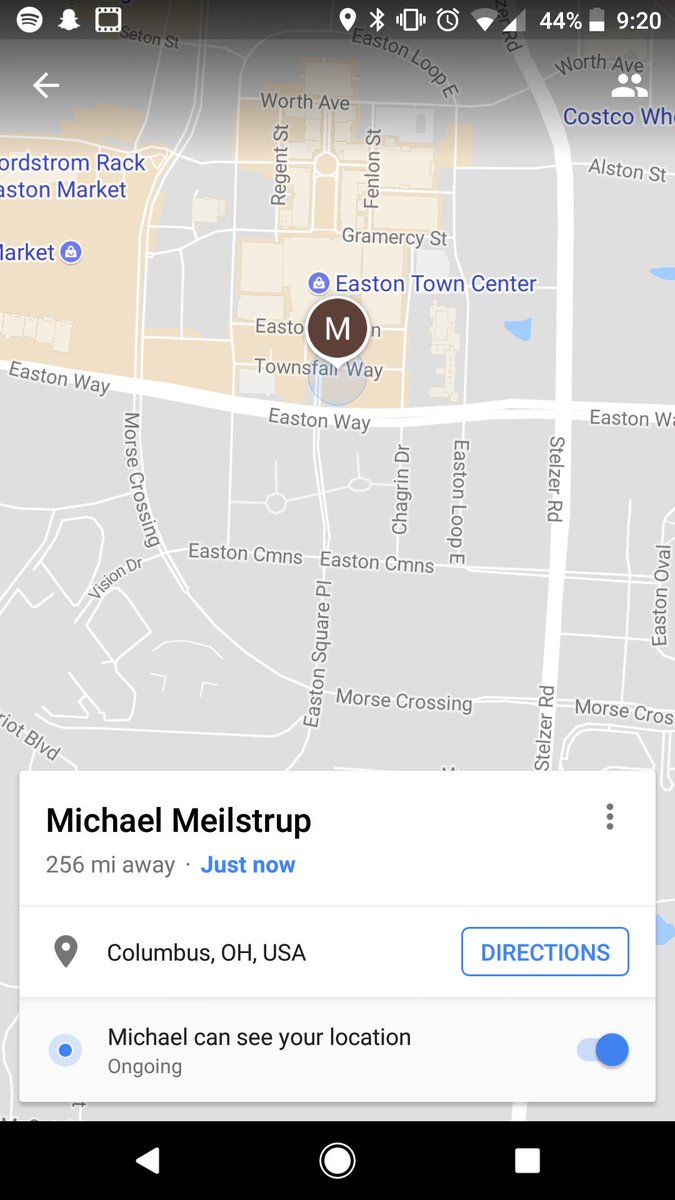This mobile device screenshot captures a detailed map-centric user interface featuring various standard icons at the top, including application notifications, Bluetooth connectivity, alarm clock, Wi-Fi connection, network connection, battery life, and the current time. At the bottom of the screen, a black rectangular box houses three navigation icons: a white backward-facing play button, a circle, and a square. The central focus of the screenshot is a close-up map of Eastern Town, indicating that the user is sharing their location. The map highlights a specific user, Michael Milstrop, who is noted to be 256 miles away, with a location pin set in Columbus, OH, USA. Additionally, there is a selected radio button confirming that Michael can see the user's location on an ongoing basis.